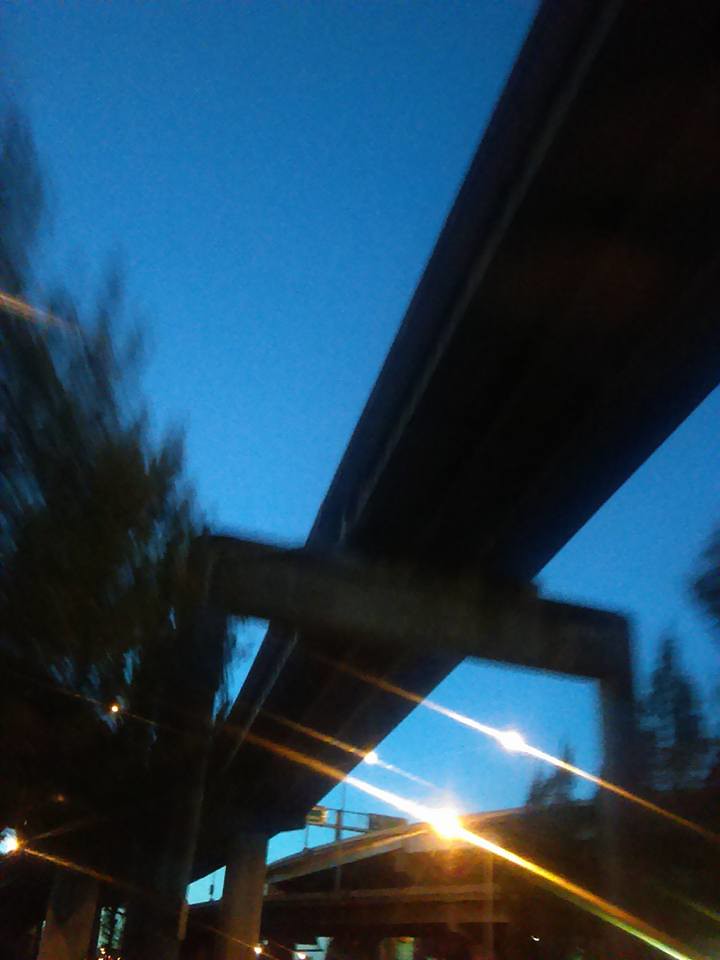A nighttime photograph captured from the ground looking upwards towards what appears to be an on-ramp or off-ramp for a highway, with the highway visible but blurred, possibly due to motion. The scene is illuminated by street lights, with the dark yet distinctly clear blue sky suggesting it’s around 7:30 or 8:00 p.m. Light flares and aberrations from the street lights are noticeably affecting the camera, creating striking visual effects in the image.